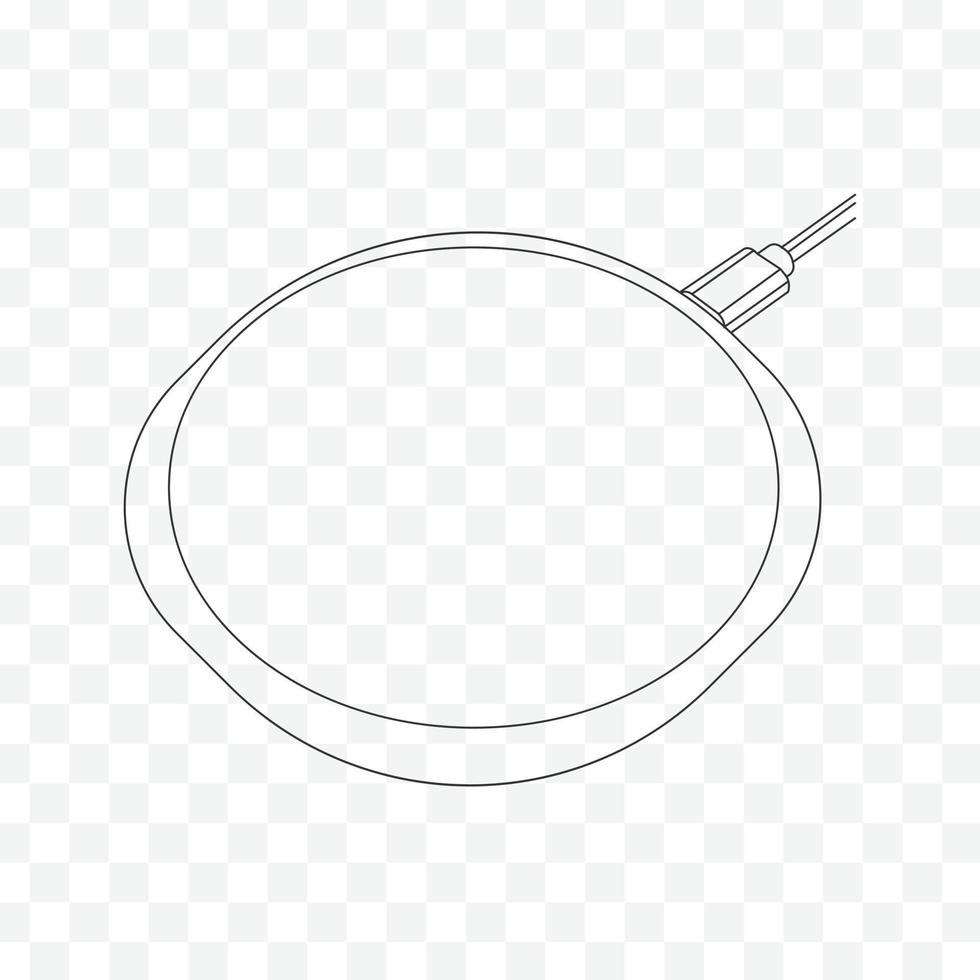This is a black line art illustration on a transparent background, indicated by the light gray and white checkerboard pattern typical of Photoshop transparency. The drawing primarily features a large circular shape, which varies in interpretation—it could represent a mirror, a magnifying glass, or a pizza paddle with an additional inner circle that might signify dough. The circular form is attached to a handle or arm, which could either be reminiscent of a wooden paddle's handle, a support arm for a mirror, or part of a magnifying device associated with drafting equipment. This handle appears to have a tapered, twisty, or elbow-like structure, suggesting functionality and maneuverability, and it’s cut off at the end. While some interpretations suggest the presence of an electrical wire, the drawing remains simple and outline-only, without intricate detailing, all set against the checkerboard pattern background.